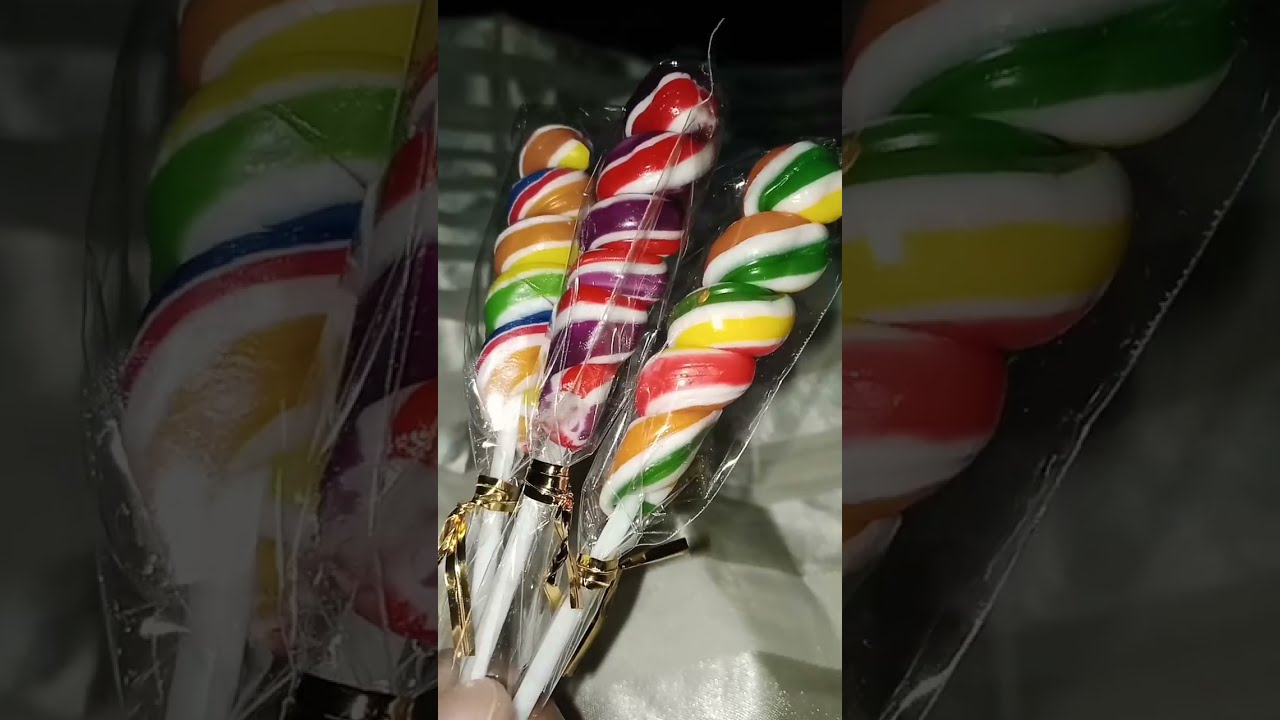The image features three vibrant lollipops held by a hand at the bottom of the frame. The lollipops are arranged in a vertical, rectangular alignment centrally positioned against a darker, blurred background of the same image, creating a layered effect. Each lollipop is encased in plastic wrap and decorated with a small gold ribbon at the base of its white stick. The middle lollipop displays a swirling pattern of purple, red, and white stripes. The lollipop on the left blends green, brown, yellow, and some blue stripes, while the one on the right combines orange, white, green, and yellow hues. The background is dark, making it difficult to discern any specific details, but the vivid colors of the lollipops stand out prominently, with no text visible anywhere in the frame. The overall effect suggests the image might be a screenshot captured from a mobile device.